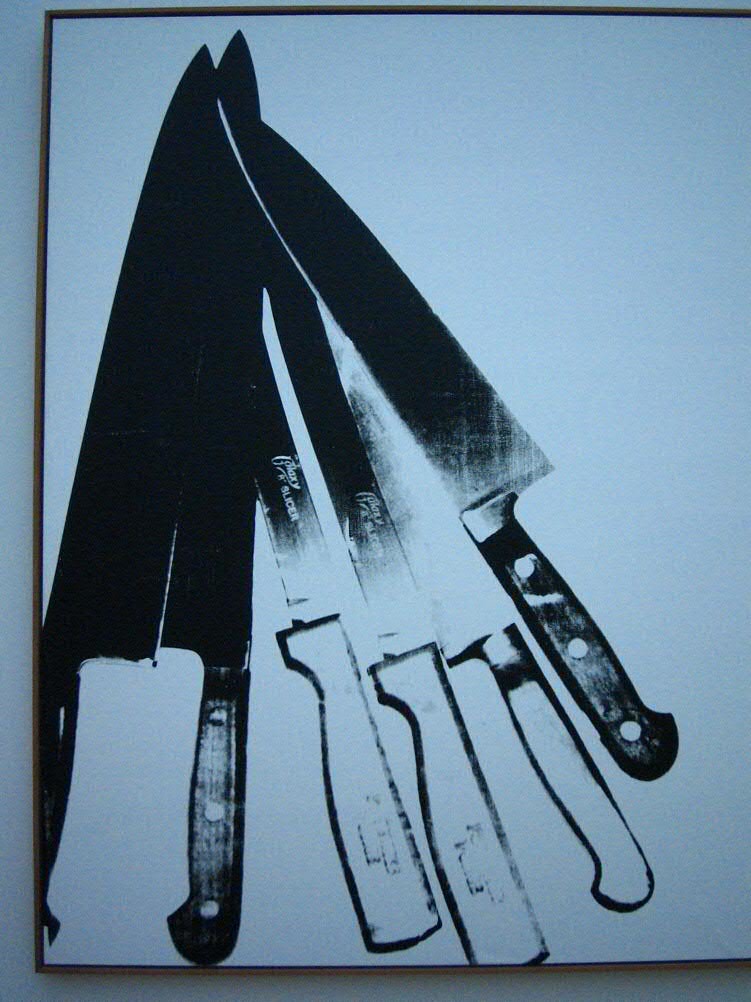The image features a light blue background with a black-brownish border forming a rectangular frame. At the center, there are six knives arranged in a visually compelling layout. These knives appear to be a mix of three carving knives and three steak knives. The carving knives have distinct black handles and dark blades, creating a stark contrast against the light blue background. The steak knives, in contrast, have handles that almost blend into the bluish tint of the background, making them appear lighter and less pronounced.

The knives are positioned facing each other in a sequential arrangement, creating a sense of movement and progression. The first knife on the left is entirely dark, including the handle and blade. As the sequence progresses to the right, each subsequent knife appears lighter, with the second knife being fully black but flipped in orientation (handle to the left and blade to the right), followed by knives that progressively lose their dark paint, especially around the handles. 

By the time you reach the far-right knife, the handle is barely outlined, and the blade appears faint, suggesting either an intentional artistic fade or the effect of decreasing layers of paint. The final knife on the left side of the image is included as if to show the source of this deterioration, with its entire surface covered in black paint, indicating that the varying darkness of the other knives is a result of the paint being worn off over time or usage.

This image uniquely blends artistic elements with a functional display of cutlery, creating a surreal and somewhat disturbing effect, as noted by the unusual painted appearances and the stark contrast between light and dark elements.